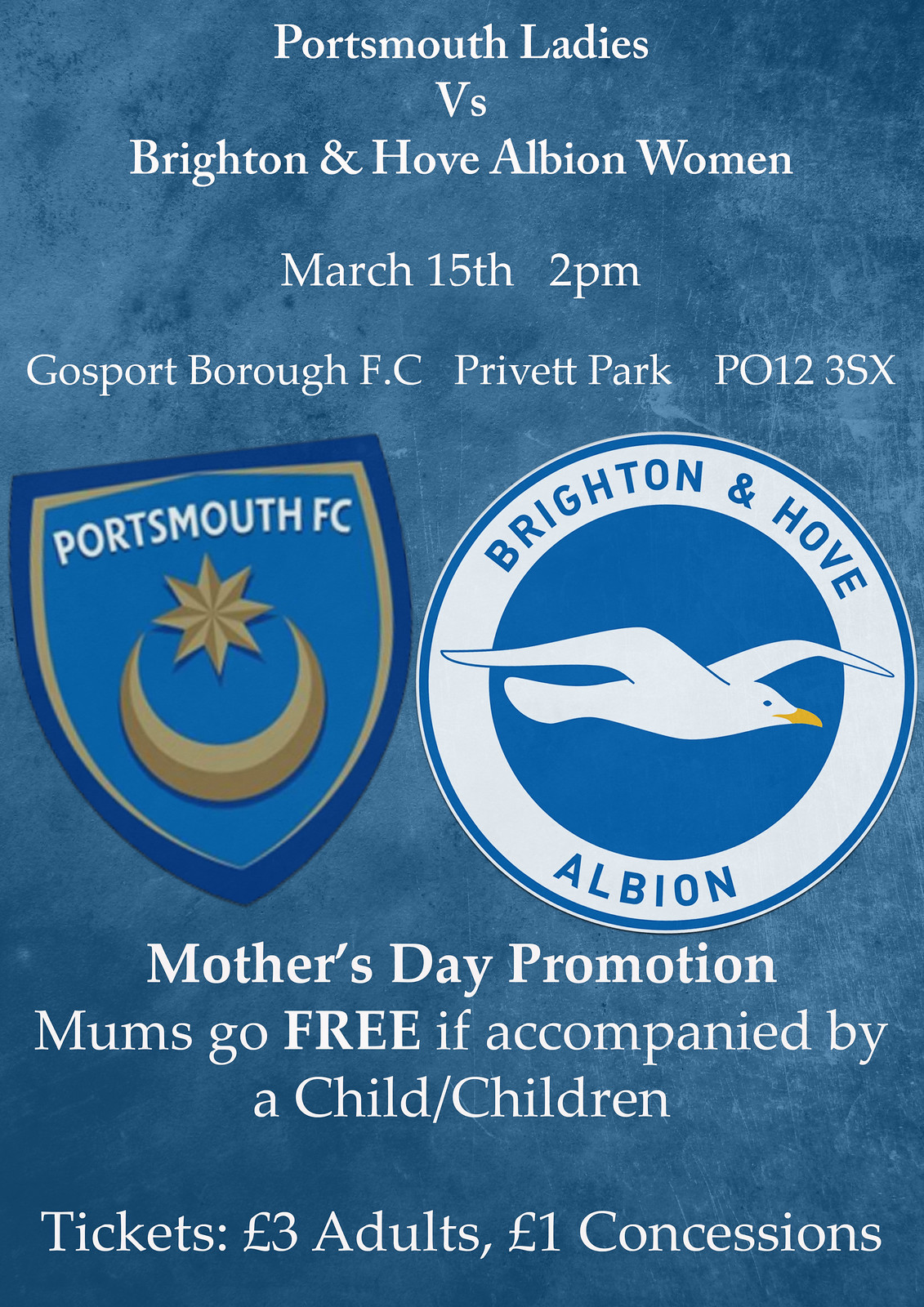This poster is for a sporting event featuring a match between Portsmouth Ladies and Brighton and Hove Albion Women on March 15th at 2 p.m. The event will be held at Gosport Borough FC, Privet Park, PO12 3SX. The background of the poster is a washed-out slate blue with a marbled texture. At the top, in white text, it says "Portsmouth Ladies vs Brighton and Hove Albion Women."

Beneath the main text, the logos of both teams are prominently displayed. On the left is the Portsmouth FC logo, which features a dark blue shield with a gold-outlined inner shield. Inside the shield, there's an eight-pointed star above a gold crescent. On the right is the Brighton and Hove Albion logo, showing a white circle with a blue inner circle containing a flying white seagull. The text "Brighton and Hove" curves around the top of the white circle, and "Albion" curves around the bottom.

Below the logos, white text advertises a Mother's Day promotion: "Moms go free if accompanied by a child/children." At the very bottom, it notes ticket prices: "Tickets: £3 Adults, £1 Concessions."